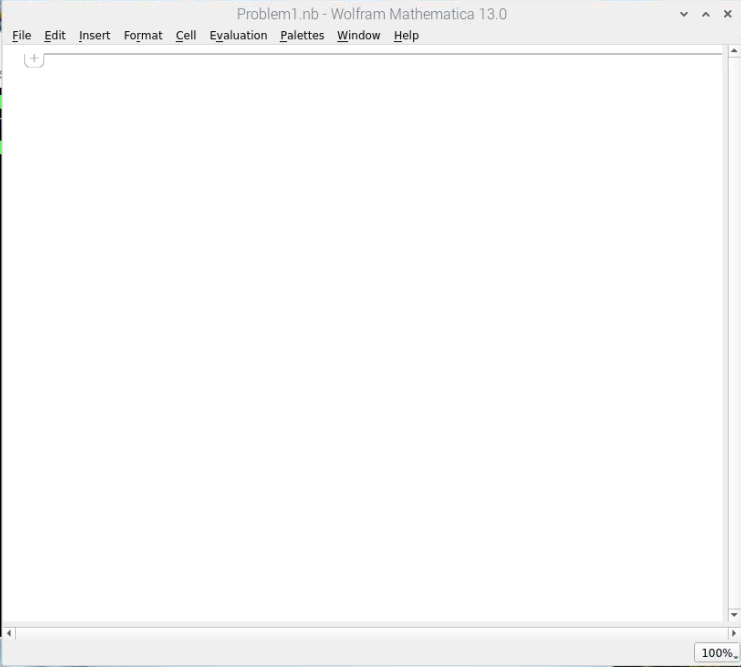A screenshot of the Wolfram Mathematica 13.0 interface, displaying a simple and clean workspace with minimal clutter. At the top, a light gray menu bar contains labeled tabs such as File, Edit, Insert, Format, Evaluation, Palette, Windows, and Help, each with their first letters capitalized and underlined. Below this menu bar, the title of the document is shown as "Problem1.nb - Wolfram Mathematica 13.0" against a gray background. The main workspace is mostly blank and white, featuring a subtle light gray plus sign indicating where new content can be added. A scroll bar is visible on the right-hand side, alongside an indicator showing "100%" in black text on a light gray background. The bottom of the interface is also gray, with the bottom center section remaining empty.